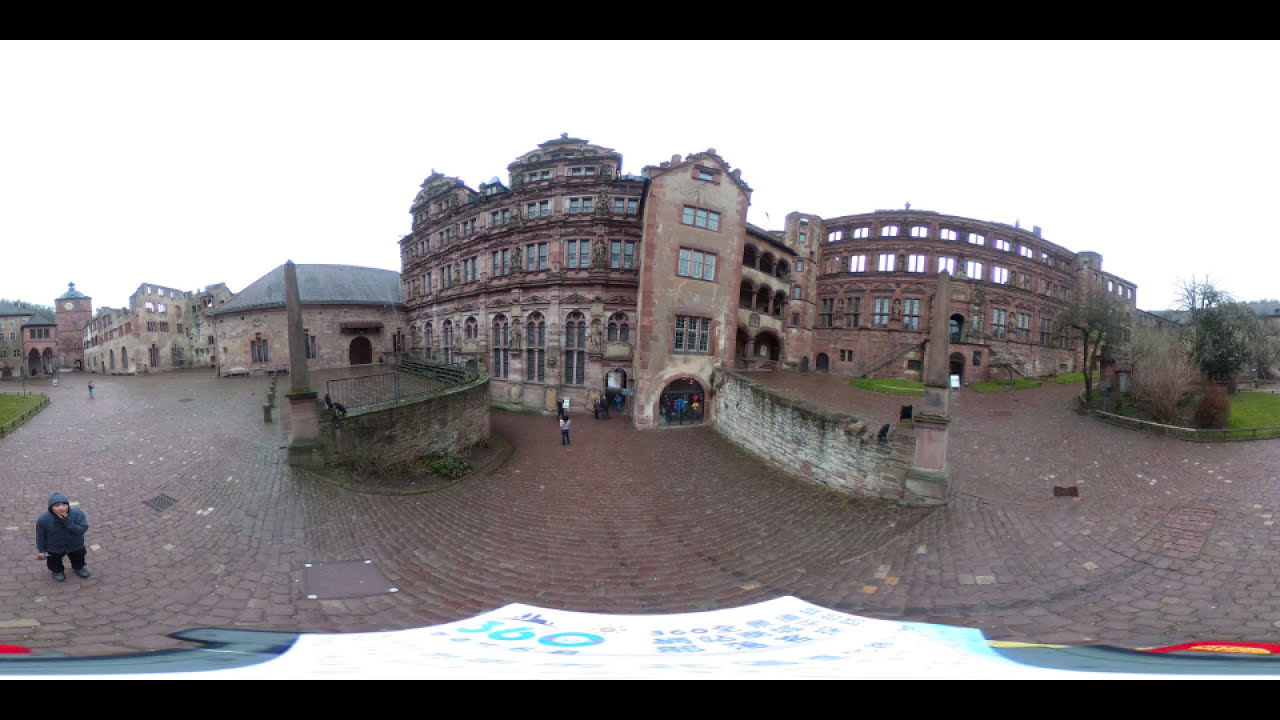The photograph captures an outdoor scene featuring a series of very old-looking red brick buildings. These structures, which might be designed in a historical or coliseum-like style, are part of a larger complex of multi-story buildings, some of them positioned on higher ground with a sloping area leading down. The sky above is hazy and cloudy, suggesting rainy or wet weather, and the cobblestone path that winds through the scene complements the rustic aesthetic of the brick buildings.

In the bottom left corner of the image stands a man wearing a blue windbreaker with the hood up, who is looking upward. The foreground also shows some small, indistinct signs with numbers and pictures, too far away to be readable. Scattered around the scene, a few more people are seen standing and observing the buildings.

There are trees and grassy patches visible, particularly on the right side of the photograph, adding a touch of nature to the otherwise industrial landscape. Despite the presence of people, the area gives off a somewhat deserted or abandoned feel, as the number of visitors is quite sparse. This detailed portrayal highlights the architectural charm and historical vibe of the setting, creating a visually engaging and interesting image.